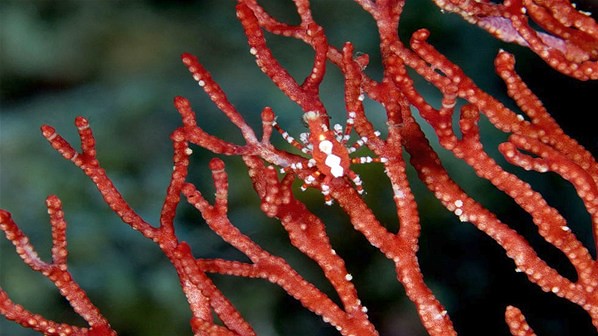This is a detailed, horizontally-aligned, close-up photographic image of a red spider camouflaged against a series of coral-like branches. The setting is outdoors during the day, and the spider appears to be almost perfectly blended with its surroundings, making it look strangely aquatic. The spider, positioned in the center of the image, has eight legs and an oval-shaped body featuring three distinctive white spots arranged in a chevron pattern. It is climbing on pinkish-red stems that branch off into smaller, shorter pieces, which have white dots on them. The background is notably blurred, transitioning from shades of green on the right to black, gray, and brown hues on the left, further emphasizing the coral and spider in the foreground. The spider's elongated and tapered head, along with its color and patterning, enhances its camouflaged appearance among the coral-like branches. The photograph, devoid of any text, captures the intricate details and natural beauty of the scene.